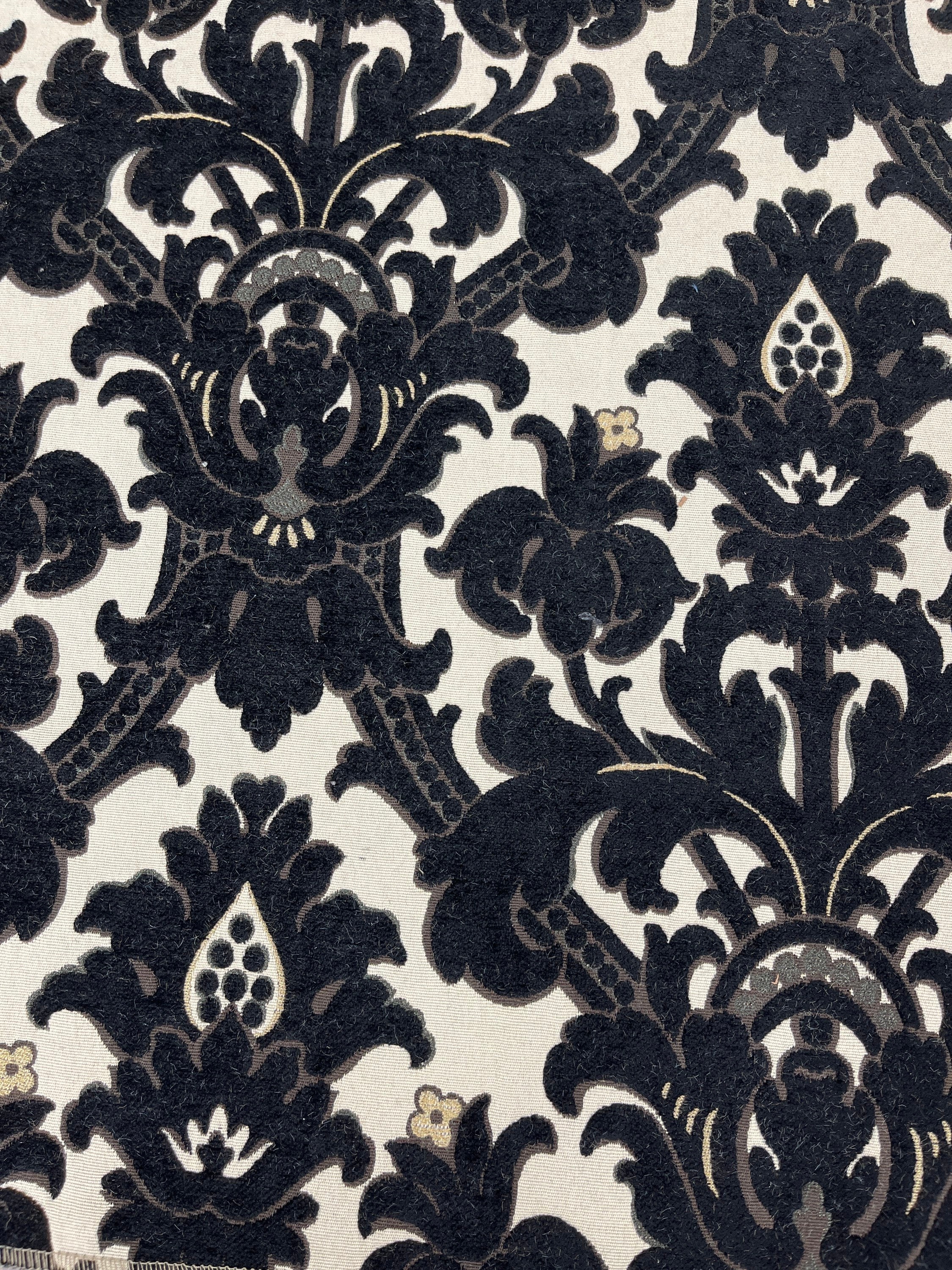This image depicts a vertically oriented pattern, potentially on wallpaper or fabric, with a highly stylized and decorative design. The predominant colors are shades of black, white, and grayscale, with accents of cream that have a slight yellowish hue. The pattern features symmetrical floral motifs, including black flowers with matching foliage, stems, and stylized feathers. These elements create a repeating tiled pattern on an off-white background. The black parts appear coarse and textured, possibly resembling felt or embroidery, contrasting with the smoother white sections that almost look cut out. There are also small gray and black ornamentations or dots enhancing the floral areas, and a slight possibility of the dark elements being an extremely subtle navy blue. The overall design exudes elegance, reminiscent of fleur-de-lis shapes, further enriched by minimalist pinstripes and diamond crossing patterns.